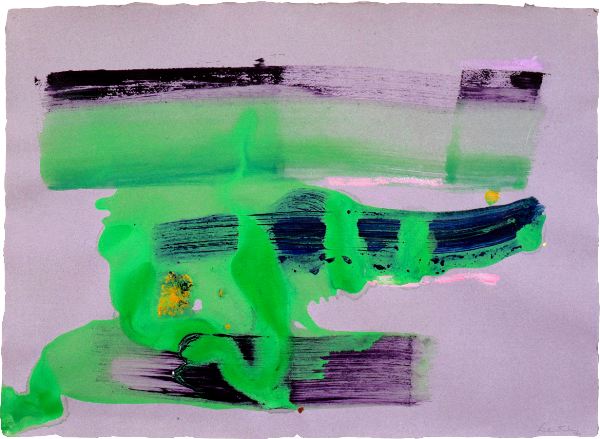This abstract painting features a dynamic composition of bold, horizontal swaths and intricate streaks of color against a lavender or lilac purple background. Three prominent black streaks run from the top to the bottom of the image, each interspersed with white highlights, and are interlaced with vibrant neon green brush strokes that suggest an almost glowing effect. The green strokes are thickest towards the bottom, with some remnants appearing to drip downwards, particularly from the middle streak, forming splotches and a small pool at the bottom. 

In the center, green paint wraps around a navy blue, shoe-like object, giving an impression of dripping fluorescence. Hints of yellow are intermixed subtly within the green, adding complexity to the composition. Further down, another streak of paint reminiscent of a strip of eggplant adds depth to the scene. Additionally, a small, distinct yellow splotch and circle appear towards the left side and in-between the top two swaths.

Overall, the painting is a mix of black, purple, and green horizontal swaths against the purple background, each infused with splashes of white and yellow, creating a rich, textured visual experience evocative of a modern, abstract style.